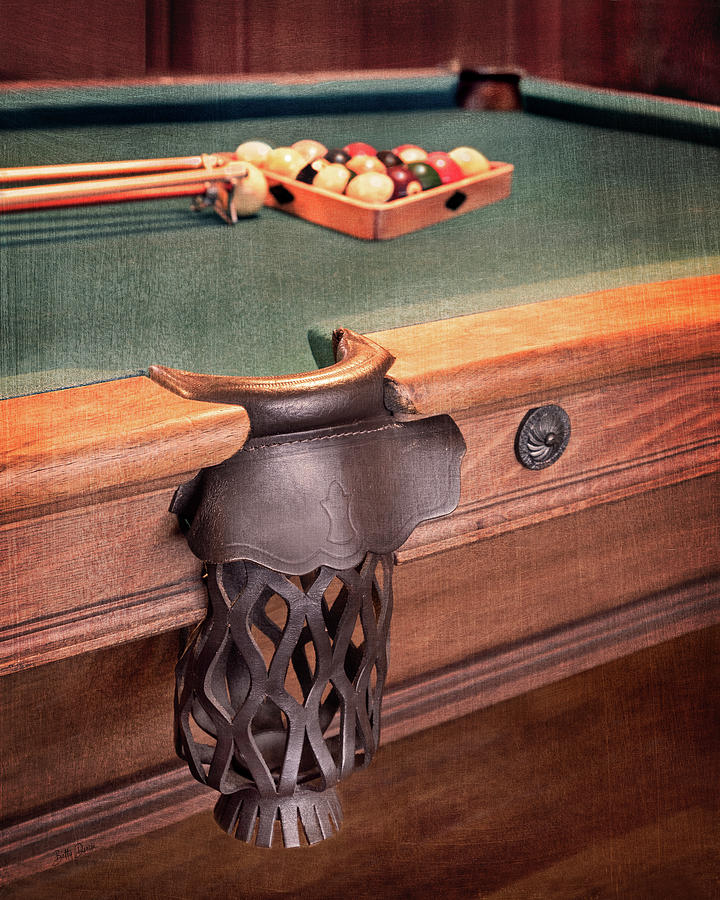The image is a color photograph capturing a side view of an old, elegantly constructed pool table. The camera is positioned along one of the longer sides, focusing on a side pocket intricately designed with woven, embossed brown leather that complements the medium brown wood of the table. This leather pocket is designed to catch the balls instead of them rolling out, a hallmark of older-style tables. The green felt surface of the table is visible, along with a wooden triangle rack filled with pool balls and two pool cues resting at the base. The polished wooden borders of the table showcase a fine wood grain, adding to the vintage charm. The setting is enhanced by a beautiful hardwood floor and wood-paneled walls, contributing to the room's traditional and elegant ambiance.